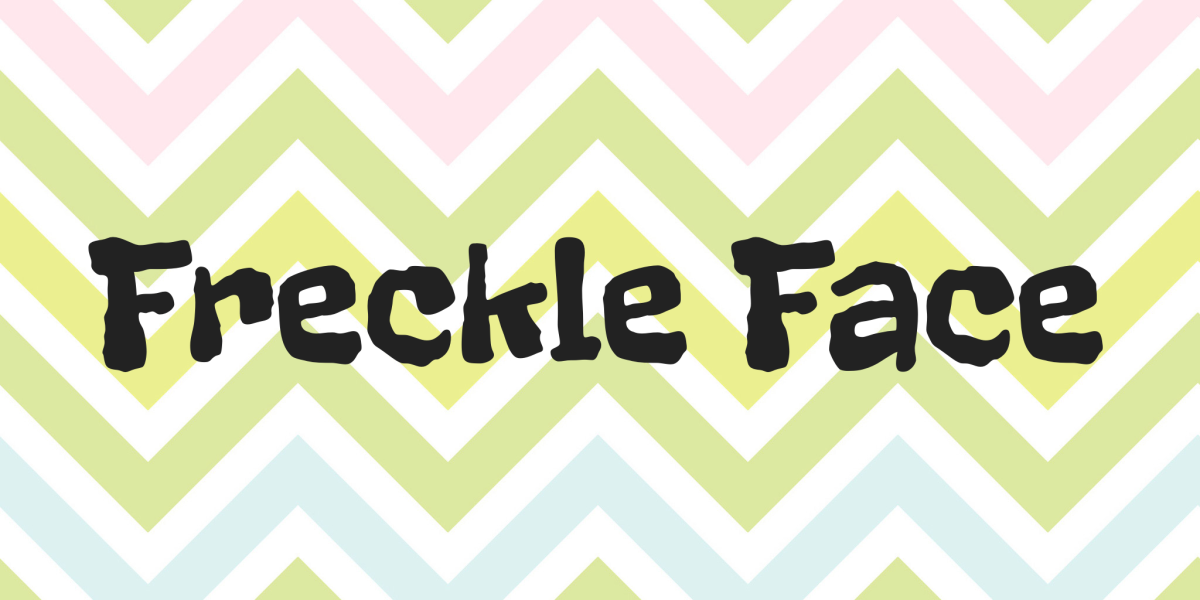The image showcases a vibrant yet slightly faded chevron pattern composed of alternating zigzag lines in pastel colors including pink, green, lime, and baby blue, separated by white lines. The chevron pattern, which features a repeating up-and-down motion, creates a visually engaging backdrop. Positioned prominently in the center of the image, the phrase "Freckle Face," spelled out as F-R-E-C-K-L-E-F-A-C-E, is rendered in a bold, black, sketchily drawn font with bumpy edges. The overall composition suggests a playful and funky design, likely intended as a logo for a brand named Freckle Face.